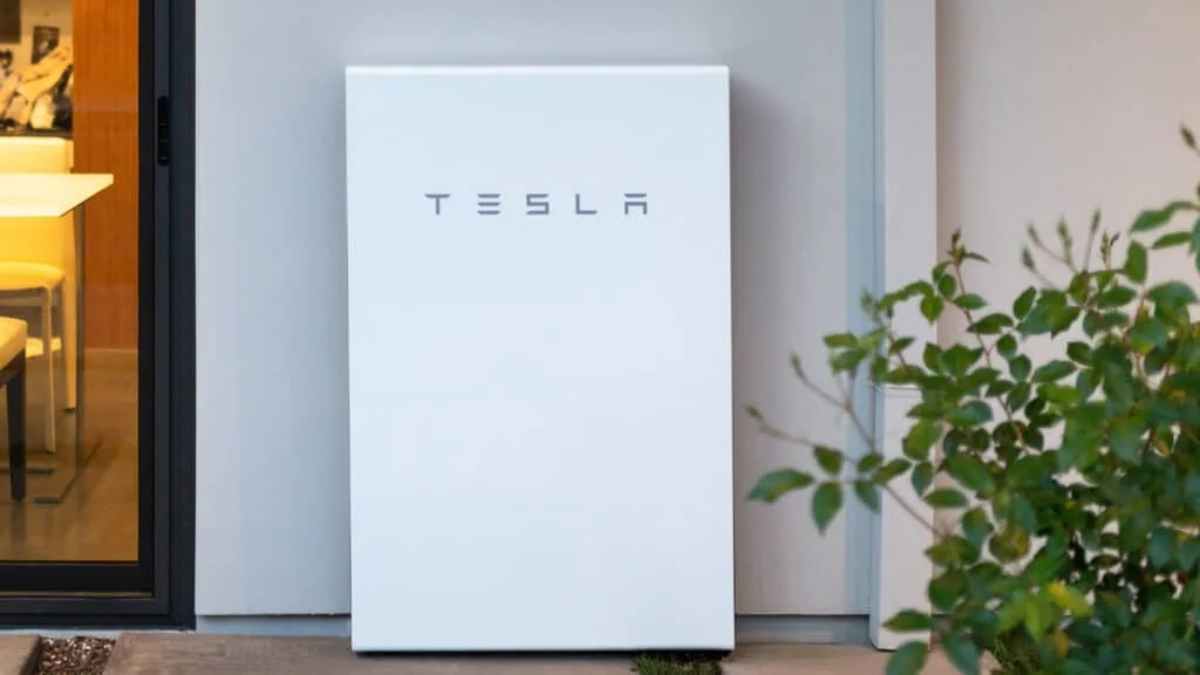The image features a striking background with a gradient of purple shades; the left side of the wall is a darker purple with a subtle blue stripe running vertically next to a prominent board. The wall adjacent to this area transitions into a lighter purple hue. In the foreground, a vibrant green plant stands out against a brown floor, which is speckled with small gold objects. A brown doorway can be seen, leading into another part of the room where a white table with a yellow chair is partially visible. Another yellow chair is also partially seen in the corner. On the floor lies a small white object. Behind this setup, there is a cabinet with a yellowish item atop it. Dominating the purple wall is a large white square panel emblazoned with the word "Tesla" in sleek, silver letters. The square panel resembles a book, with a glint of gold color peeking from under its edge, adding a touch of elegance to the overall composition.